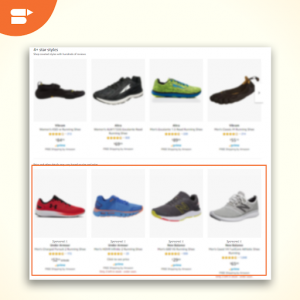This screen grab depicts a section of a website, featuring a compact display measuring approximately two inches by two inches. Dominating the top left corner of the page is an orange logo, which consists of a white emblem resembling an 'S' formed by two bars and an arrow pointing to the right. The logo itself lacks any accompanying text to identify the company.

Central to the image are eight pairs of shoes arranged in two neat rows of four. These shoes appear to cater to running, walking, or other sports-related activities. Although the accompanying text is largely unreadable, it is evident that each pair of shoes is accompanied by a rating, a price, and a possible brief description beneath it.

The website interface in the image is set against a light yellow background with the main page being predominantly white. The shoes are displayed against a subtle light gray backdrop. Notably, the second row of four shoes is distinctly highlighted with a red or orange border, drawing particular attention to these pairs.

The varied shoe selection showcases a spectrum of colors including black, green, blue, white, red, yellow, and various shades of gray. Among the predominantly athletic footwear, there are also one or two pairs of black sandals.